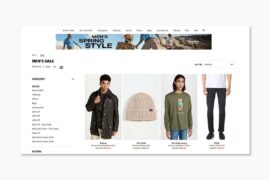The image depicts a webpage from an e-commerce clothing website, showcasing a diverse range of apparel. Prominently featured is a black button-down shirt paired with tan pants, and a beige beanie. An olive green t-shirt with a logo is also visible. Additionally, there is an outfit consisting of a white shirt and black pants. The webpage is designed with a clean, predominantly white background and black text, providing various text options for filtering selections. At the top of the page, a banner ad titled "Spring Style" displays assorted outfits worn by models in natural, seasonal settings. The layout and text elements suggest a typical user interface for browsing and purchasing clothing items online.